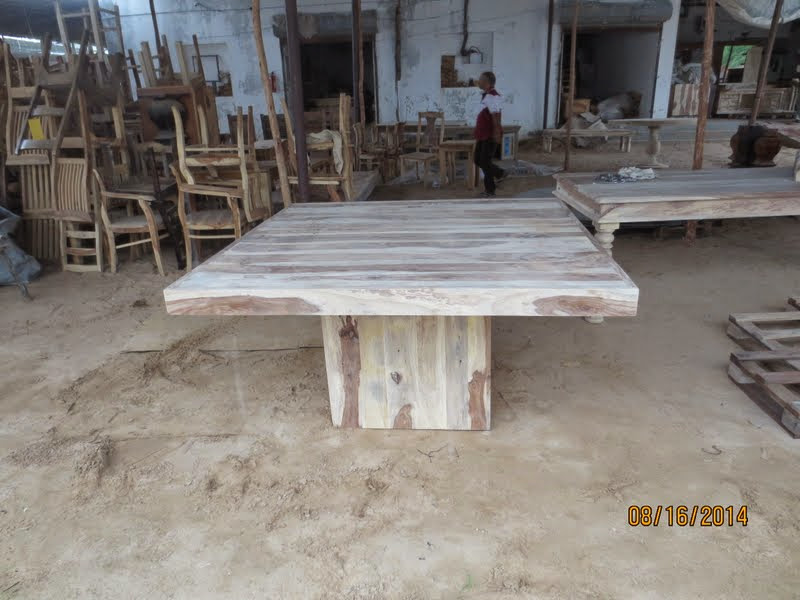This image depicts an old, partially open woodworker's shop or warehouse with a distinctive rustic ambiance. The foreground features a large, unfinished, wooden workstation table with dark brown spots and a visible platform underneath. Adjacent to it, on the right side of the frame, is a wooden table with four legs, accompanied by two wooden crates. 

Prominently in the center of the image, a man dressed in black pants and a red-and-white striped shirt is walking towards the left, but his details are indistinct. The date "08-16-2014" is marked in orange or gold at the bottom right of the image, likely indicating when the photo was taken.

The background to the left is cluttered with a myriad of wooden chairs—dining, kitchen, and living room chairs—piled haphazardly, some stacked, some upside down, and all unfinished. Numerous pieces of furniture, including dressers, headboards, a round dining table, low coffee table, and a bar or counter, are dispersed throughout the scene, all awaiting final touches.

The workshop's walls are white but marred with peeling paint, and the floor appears to be a grayish-brown concrete with dirt patches. The storage areas in the back seem to shelter finished products, prepared for shipping. While no woodworking equipment is visible, suggesting this is a finishing area, the setting communicates a sense of industrious activity within a large, pavilion-like structure.